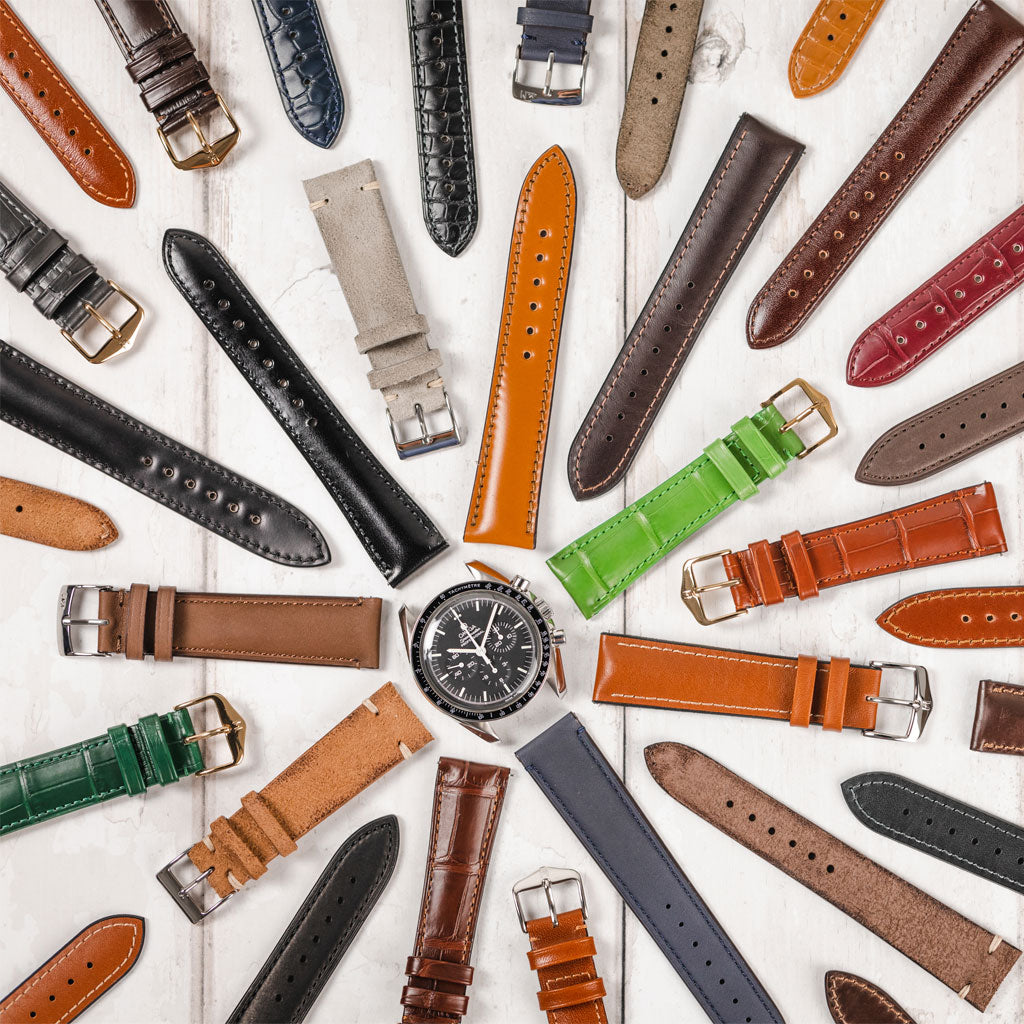This product demonstration image showcases a high-end watch prominently situated just below the center point of the photograph. The watch is distinguished by its silver, platinum, or chrome metal casing, featuring a black dial with a black and white color scheme. This intricate watch face displays not only regular time-keeping elements such as minutes, hours, and seconds but also additional functions that may include a date setting, secondary time zone, and potentially a compass. Although the precise details of the watch face are somewhat difficult to discern, the central importance of this image lies in illustrating the versatility of interchangeable watch bands.

Surrounding the unattached watch face, arranged in a star-like circular formation, are numerous watch bands showcasing a variety of colors, patterns, and textures. Closest to the watch face, there are leather bands in shades of black, gray, and three different browns positioned on the left and right. Two orange bands and one bright green band add vibrant color to the initial circle. Extending outward from this central array are additional bands in tan, blue, red, orange, and green hues, as well as some with intriguing animal skin patterns resembling alligator or snake.

This layout emphasizes that the watch can be customized with a broad range of bands to match different outfits and occasions, highlighting its versatility. The presence of unique bands, such as one in lime green, further underscores the wide array of stylistic choices available. Although the styles and colors suggest a feminine aesthetic, the design also retains a unisex appeal. Overall, this image effectively communicates the concept of a customizable watch suited for those seeking both functionality and personalized style.